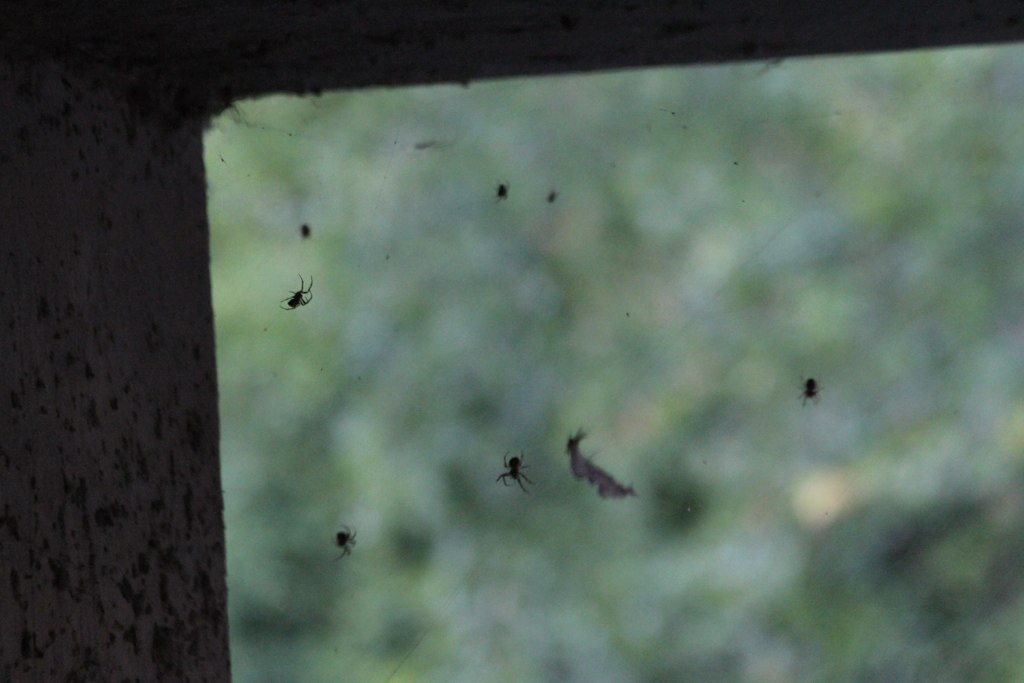This is an image displaying numerous spider webs with several spiders prominently featured. The scene seems to be viewed through a window, which might belong to a garage or basement, as indicated by the grayish wall and ceiling on the left and upper portions of the image. The background is a blurred mix of green and yellow hues, suggesting distant foliage or trees, though no details are discernible. Despite the faint lines indicating the presence of cobwebs, the intricate details of the webs remain obscure. However, the spiders are clearly visible, with around seven in total, including both sizable and small ones, scattered about the window. Some of the spiders appear to have caught something in their webs, and while the window structure is apparent, the outside view remains largely a green, indistinct blur.